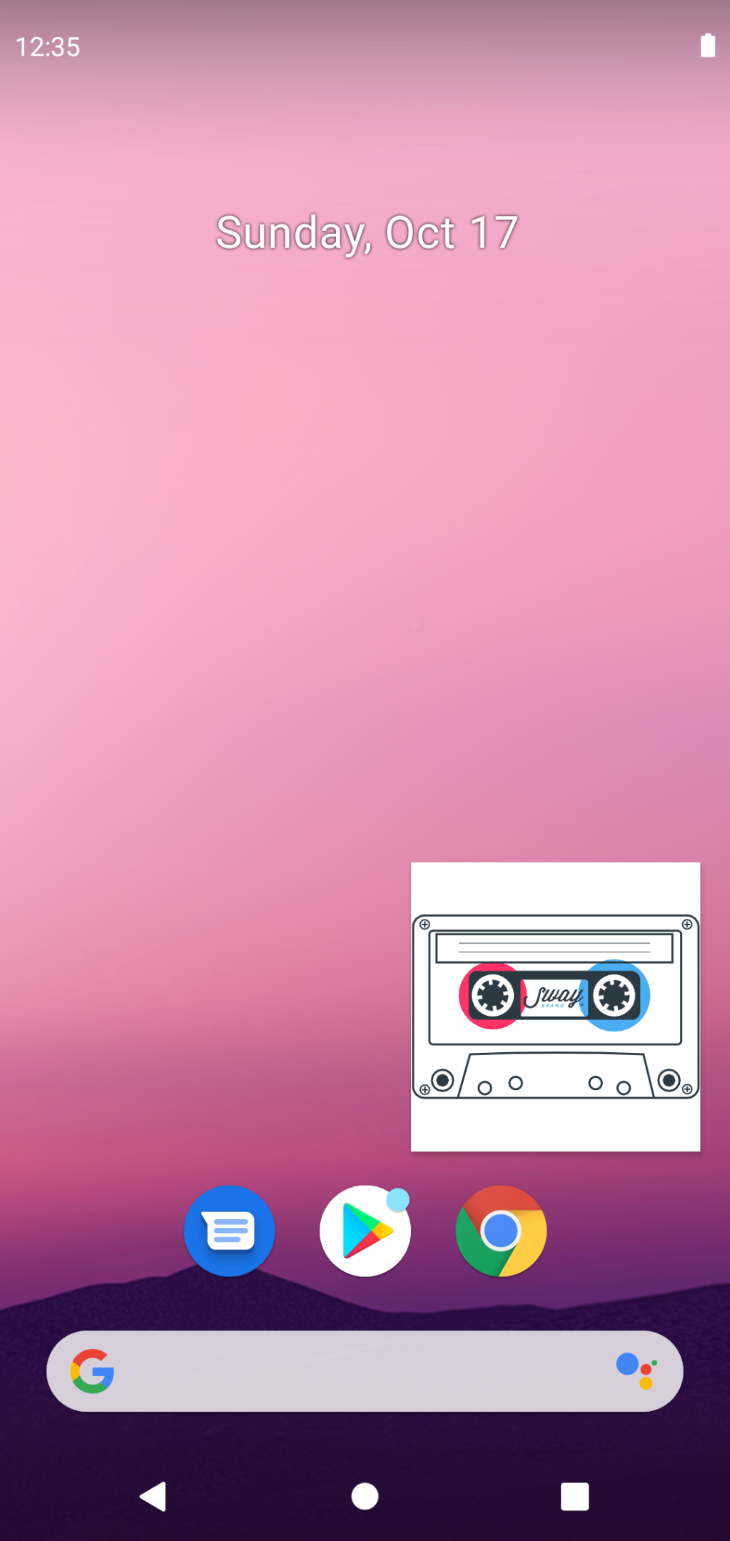This is a detailed screenshot from a smartphone. In the top left corner of the screen, the time is displayed as 12:35. The top right corner shows a nearly full battery icon. Central to the screenshot is the date, prominently displayed as "Sunday, October 17th." The background features a gradient starting with dark purple at the top, transitioning into pink, and gradually darkening again to hues of pink, purple, and almost black. In the middle of this gradient background, there's a hand-drawn image of a cassette tape. Below this image, three website icons are visible, starting with the Google Play Store, followed by Google Chrome, and a Google Search bar beneath them. In the bottom left corner, there's an arrow pointing left, and next to it is a small round circle, which is the Google app icon. At the very bottom, the gradient starts as dark purple and fades seamlessly into light pink.